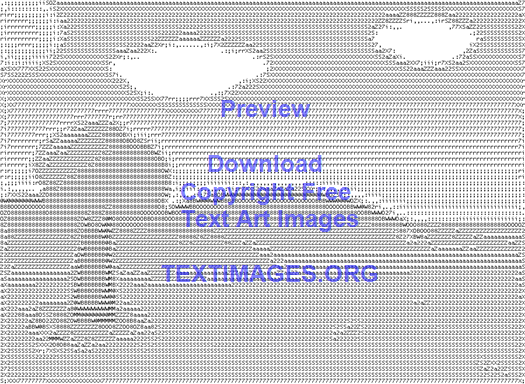This computerized art image portrays a detailed scenery made entirely of numbers and letter characters. Upon close inspection, one can see the intricate arrangement of various characters such as '2's, 'S's, 'O's, 'B's, and 'M's, creating a cohesive picture. The scene features a grassy ground with a prominent tree, overlaid by a sky dotted with clouds. The characters, primarily in green, are set against a white background, adding depth through varied character density, which creates darker and lighter areas. In the center of the image, there is purple text that reads "preview download copyright free text art images textimages.org," likely edited in post-production. This elaborate arrangement of keyboard characters seamlessly forms the natural elements, blending both art and text.